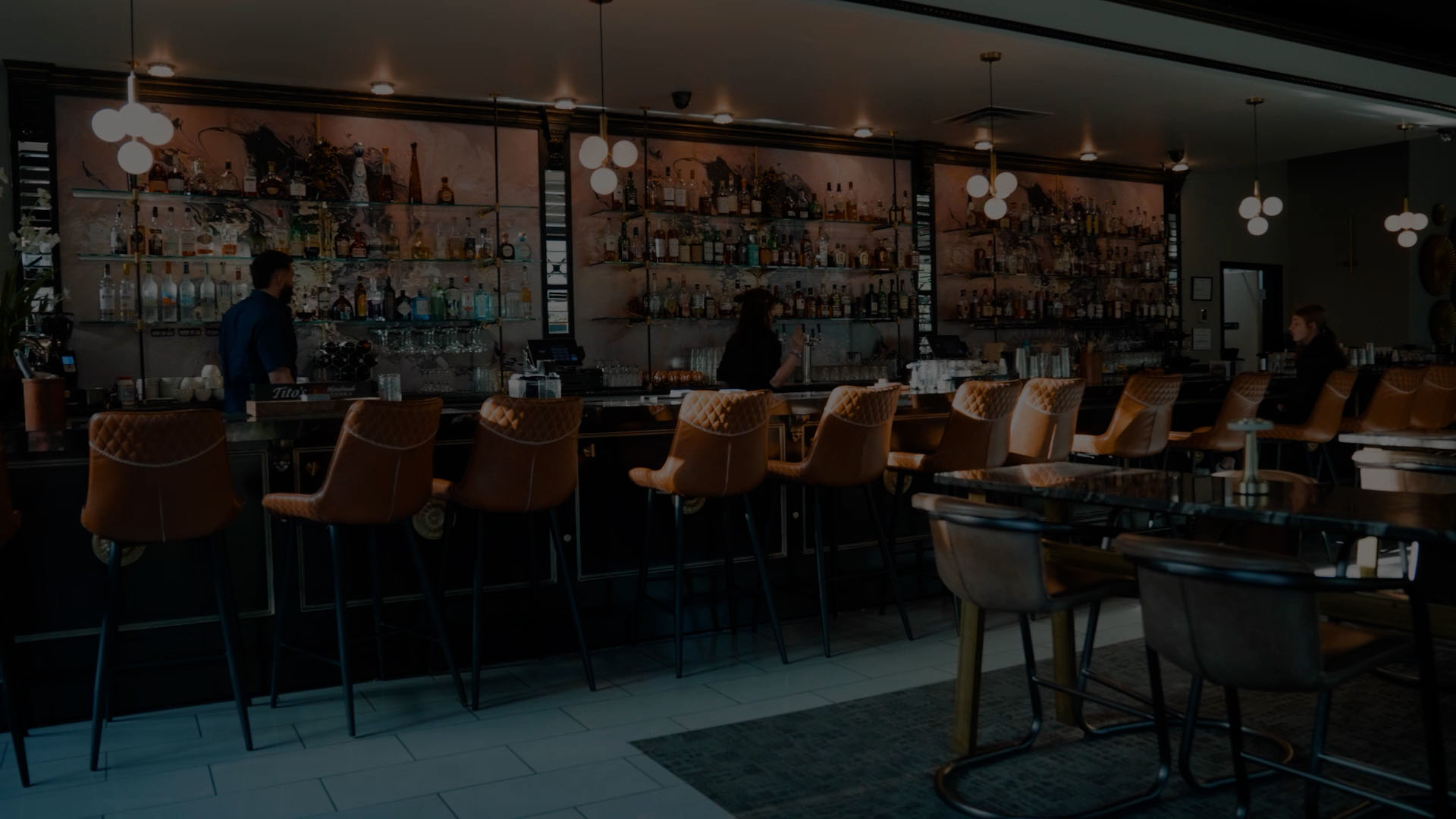The image is a dimly lit photograph of what appears to be a bar setting in a restaurant that isn't currently open. The rectangular, horizontal frame captures a space featuring a mix of table seating and a bar area. Along one side of the wall, there is a row of tables with dark, reflective surfaces surrounded by chairs.

In the right corner stands the bar, which is highlighted by several features: it has shelves stocked with various bottles of liquor set against a white background that creates a striking contrast. The bar is fronted by about ten orange-colored, leather-looking stools with backs, appearing lighter brown in the faint light. Some stools might be occupied, but the darkness makes it difficult to discern details. 

The ground is covered with light gray, large-tiled flooring, resembling a brick pattern. Above, multiple lighting features exist, though they aren’t fully illuminated. Globe lights line the top of a wood-paneled wall while sets of three pendant lights hang from the ceiling, with additional recessed lighting creating a soft ambiance.

Despite the low light, you can vaguely make out a bartender, and possibly another person, behind the bar, though they remain indistinct due to the darkness. The overall composition and subdued saturation give the scene an atmospheric, almost mysterious quality.